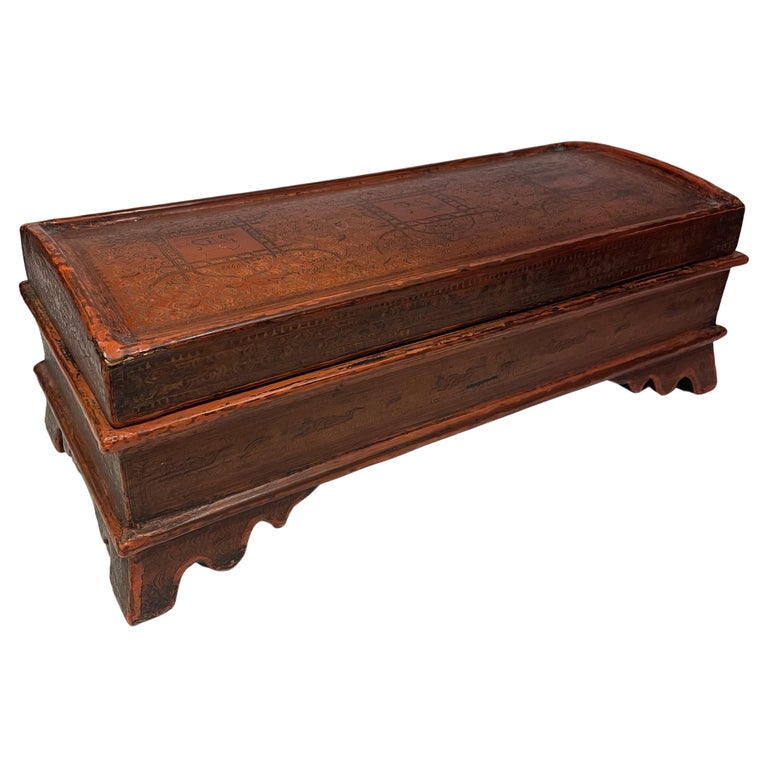This image is a detailed color photograph of an antique, dark brown wooden chest displayed against a clean, white background. The chest has a rich, shiny finish and exudes a vintage charm, suggesting it could be over a century old. It is rectangular in shape with four sturdy legs that feature graceful, inward-curving lines and squared corners. The bottom of the chest is accented by a recessed edge; just above it, there is a prominent lip that runs around the piece. This lip is echoed at the upper part of the chest, where a slightly curved lid sits atop. 

The lid, which likely functions as a removable top for storage, showcases intricate, old-world graphic designs, possibly resembling a shield with ladder-like patterns along the sides. Despite its elegant design, the chest bears some signs of wear and tear, indicating its age and use over the years. The entire piece is constructed from thick, hefty wood and appears quite solid. The photograph isolates this antique artifact, allowing its rich details and craftsmanship to stand out against the stark, white background.